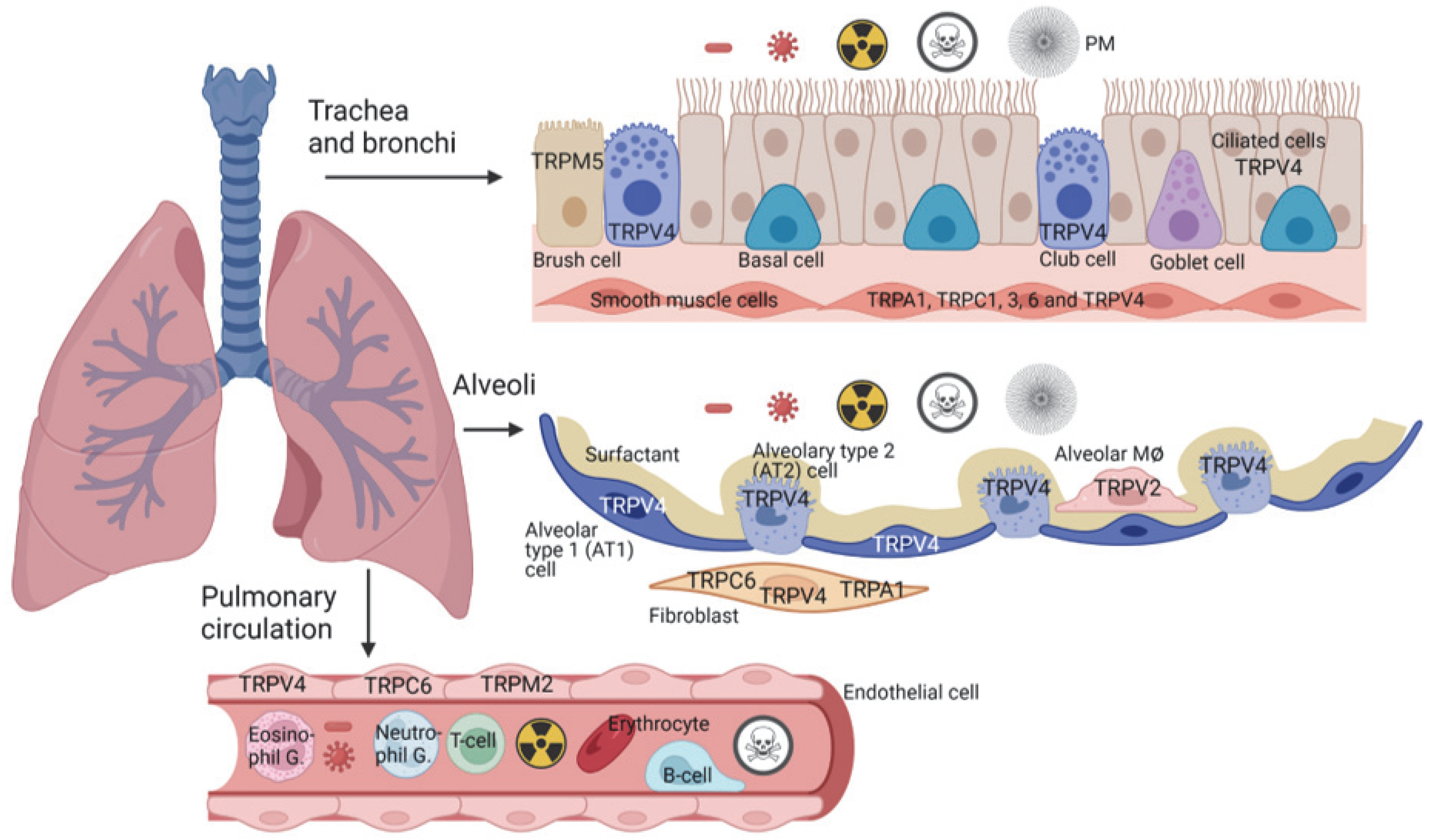The animated image presents a detailed visualization of various parts of the respiratory system and certain cell types. On the left side, prominently showcased, are the two pink lungs. Intricate networks of purple veins or bronchi branch throughout the lungs. A black arrow points to the right lung with a label reading "Pulmonary Circulation." 

Additionally, the animation features a complex depiction involving T-cells and other immune cells, integrated into the broader respiratory context. The respiratory lining sees a microscopic view, illustrated with floral-like structures. Scattered throughout are labeled cells, including breast cells, facial cells, club cells, goblet cells, and smooth muscle cells, emphasizing their diverse roles in lung and respiratory function.